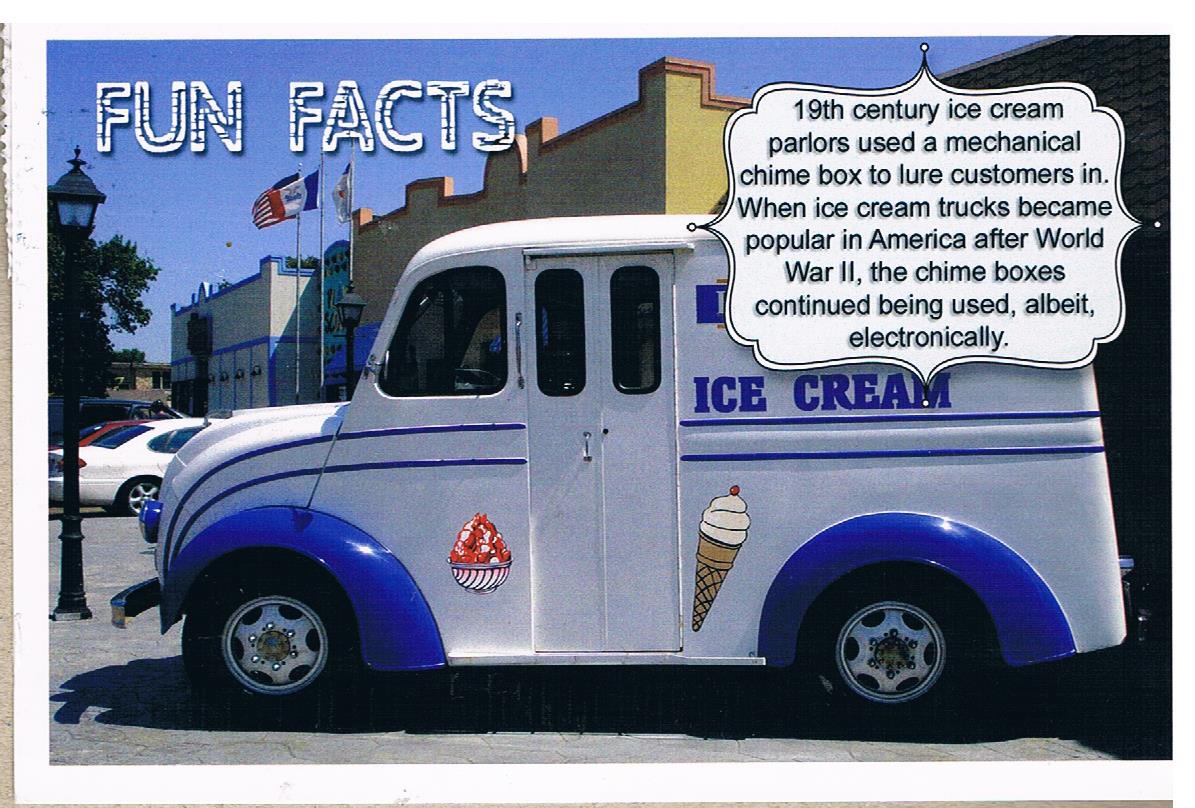The image is a vintage postcard placed on a tan-colored table, showcasing an old-fashioned ice cream truck parked in front of sandstone buildings with flags and a lamppost nearby. The postcard has a white border with a slight tan margin visible along the left side and bottom. The ice cream truck, which has a light blue tint and dark blue accents, features large blue fenders, blue pinstripes, and signs displaying ice cream cones and a sundae. The truck's side bears the text "Ice Cream." In the top left corner of the postcard, white text reads "Fun Facts," while the top right corner holds a stylized information box with black text, stating: "19th-century ice cream parlors used a mechanical chime box to lure customers in. When ice cream trucks became popular in America after World War II, the chime boxes continued being used, albeit electronically."